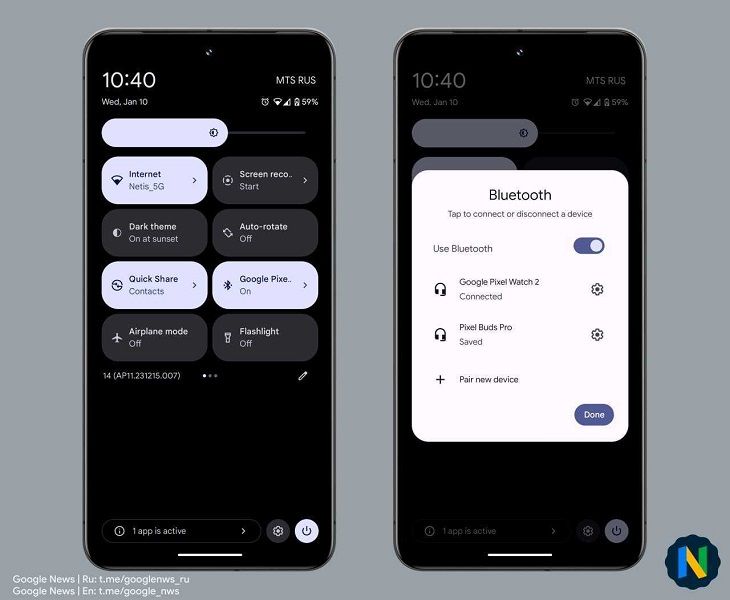This image features a side-by-side comparison of two smartphone screens, displayed prominently against a plain grey background. The phone on the left shows a screen with the date and time: Wednesday, January 10th, at 10:40 AM, along with a battery level of 59%. The screen displays various quick settings such as Internet, Screen Recording, Dark Theme (enabled), Auto Rotate, Quick Share, Google Pixel, Airplane Mode (disabled), and Flashlight (disabled).

The phone on the right highlights Bluetooth settings, showing an active connection with a Google Pixel Watch 2 and saved pairing with Pixel Buds Pro. Users are prompted to "Pair a New Device" and have the option to "Done" when finished. This phone screen is likely part of a Google News article intended to guide users through connecting devices via Bluetooth.

Both phones' backdrop features a grey hue, with minimal distractions. At the bottom left of the image, the Google News trademark stamp is visible, indicating the source of the information. On the bottom right, there is a logo resembling a blue circle with blue, yellow, and green elements, reminiscent of Google's branding.